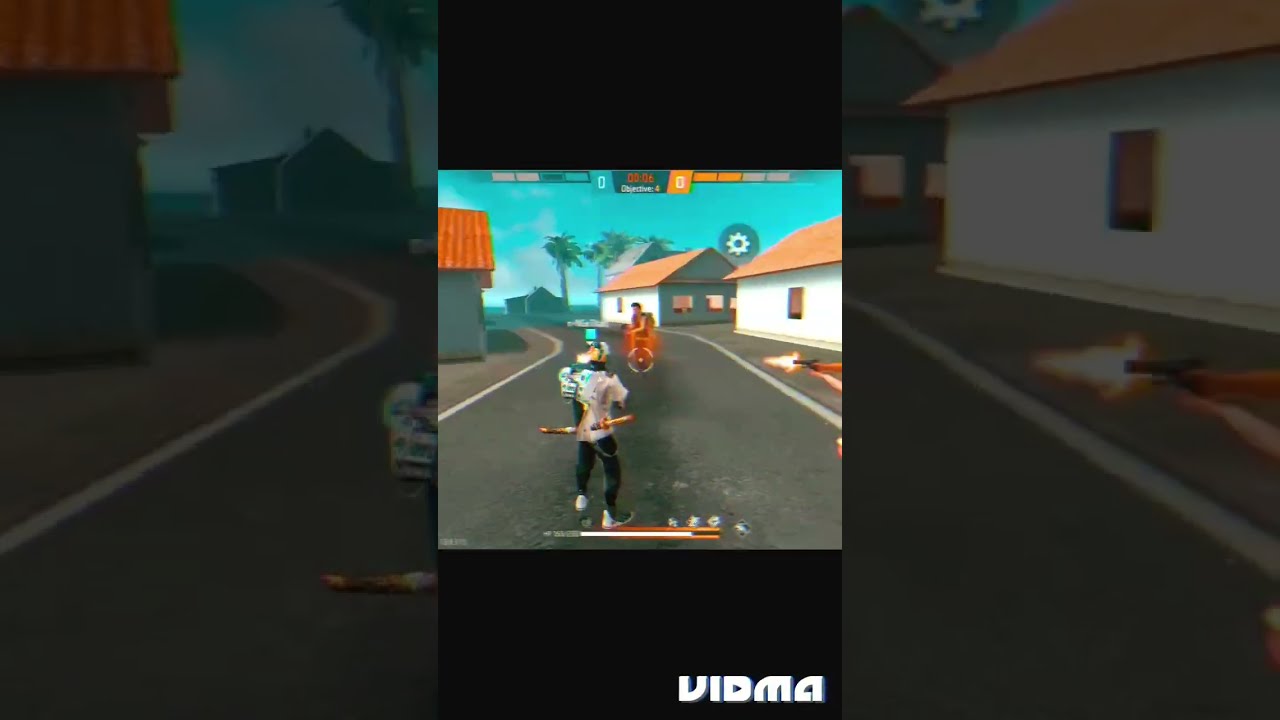This image is a horizontal rectangle divided into three panels, with the left and right panels forming the background and the middle panel superimposed over it. In the left panel, the scene depicts a street curving to the left with a building on the left and another building with a tree beside it in the distance. The right panel shows the opposite side of the same street, featuring several buildings and two arms holding a firing gun, indicated by red and white lights at the gun barrel. The central superimposed panel, bordered in black at the top and bottom, mirrors this street scene but adds additional elements, including a character with a sword on his back walking down the street, accompanied by an indistinct figure ahead of him. The middle of the scene shows a shooting reticle, hinting at gameplay, and various trees, small white houses, and a sky are visible in the background. The video game interface's display, including a settings icon and the text "VIDMA" at the bottom, suggests a basic 3D third-person shooter game, possibly on a mobile platform. The color palette includes shades of gray, white, orange, brown, green, and blue, typical of a video game screenshot akin to Fortnite.